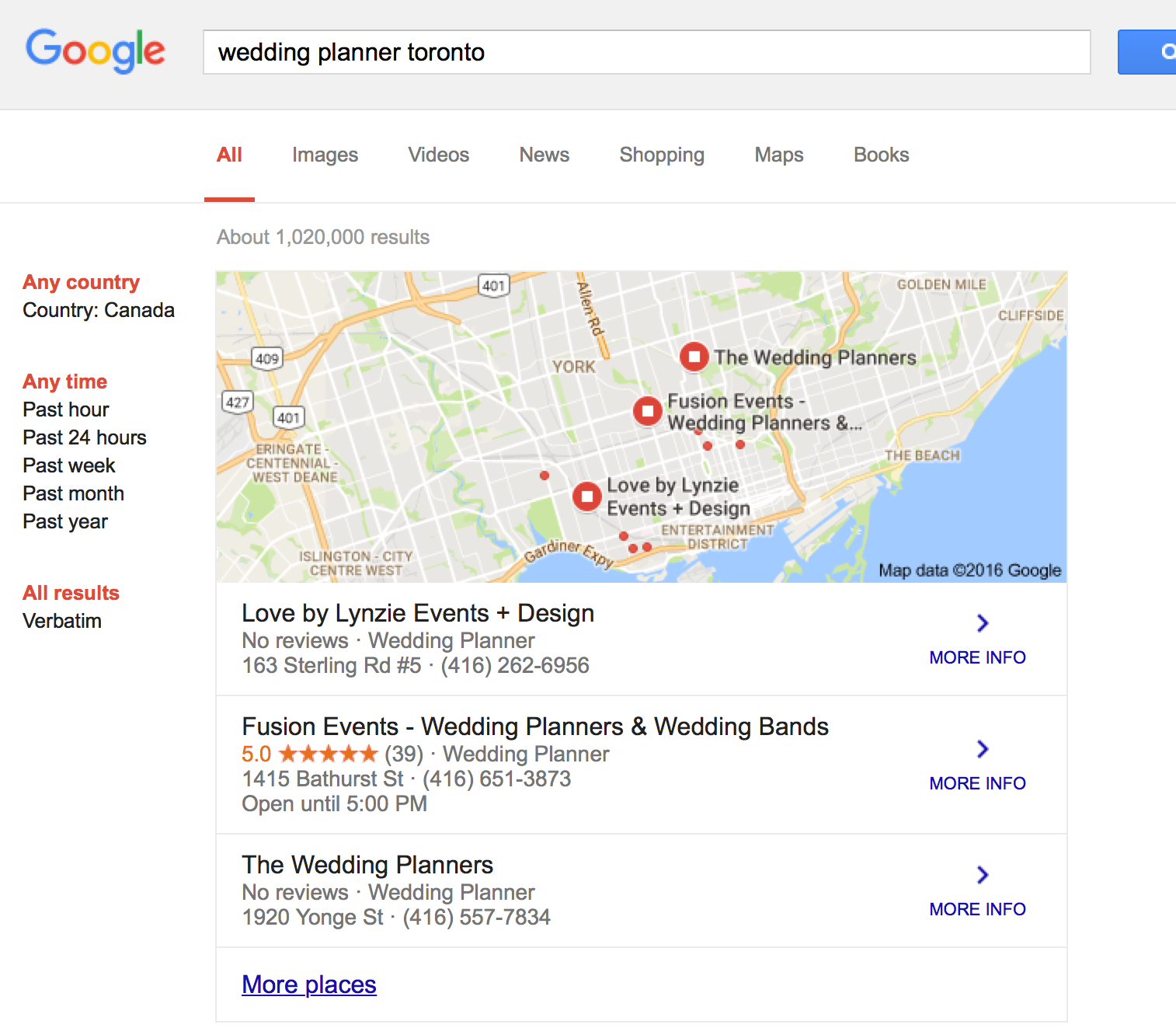The image captures a Google search page for "Wedding Planner Toronto," displayed on a clean, white background. In the upper left corner, the iconic Google logo in blue, red, yellow, and green is prominently visible. The search box in the center reads "Wedding Planner Toronto," and to its right sits a blue button with a white magnifying glass.

Directly below the search bar, a red underlined tab labeled "All" is visible, alongside gray tabs for "Images," "Videos," "News," "Shopping," "Maps," and "Books." The search yields approximately 1,020,000 results. An image of Toronto cityscape is captured below, featuring numerous markers highlighting different wedding planners’ locations. The highlighted entries likely represent those who have invested in Google’s advertising services, as indicated by larger red markers, contrasted with smaller red dots for other planners.

Three prominent wedding planner listings are displayed:

1. **Love by Lindsay Events and Design**: No reviews. Listed under "Wedding Planner" with accompanying address, phone number, and additional information.
2. **Fusion Events Wedding Planners and Wedding Bands**: Highly rated with a 5.0 score from 39 reviews. Listed under "Wedding Planner" with address, operating hours, and more info.
3. **The Wedding Planners**: No reviews. Listed under "Wedding Planner" with contact information and more details.

A hyperlink for "more places" offers additional options beyond the highlighted entries. On the left sidebar, filters include options such as "Any country," with "Country Canada," various time-frame selections, and a choice for "All results verbatim."